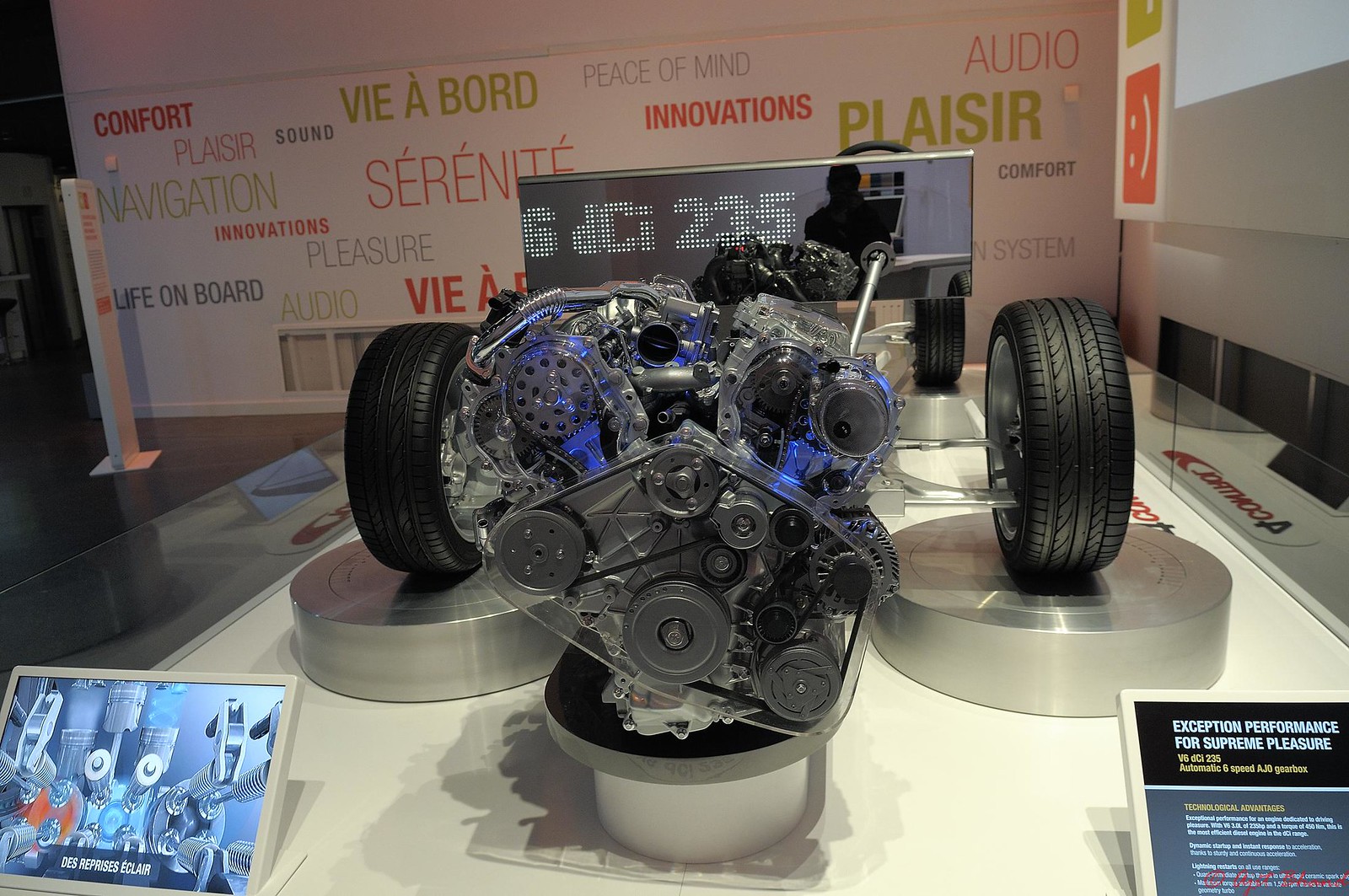The image depicts a detailed model of a drag racing car with a large engine centrally located, flanked by two prominent black wheels. The vehicle appears to be elevated on stilts in a brightly lit room with white walls. Various signs are displayed on the wall behind the car, with words in both English and other languages. Visible English words include "comfort," "audio," "innovations," "sound," "peace of mind," "pleasure," "life on board," and "navigation." Additionally, behind the engine, a display board presents characters and numbers such as "C," "D," "C," "I," "2," "3," and "5." At the bottom right corner of the display, text reads, "exception performance for supreme pleasure." This scene suggests an environment like a technical school, exhibition, or design studio, showcasing the clean and innovative aspects of the car model.